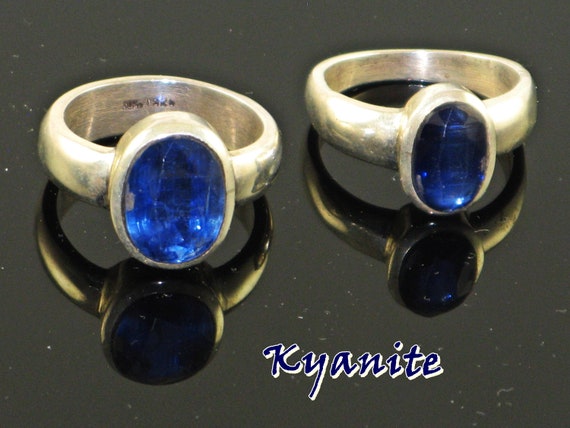This is a detailed photograph of two rings positioned side by side on a reflective, charcoal gray surface. The surface flawlessly mirrors the rings, adding depth to the image. The rings, which bear a striking resemblance, are made from a material that looks like sterling silver. The one on the left is slightly larger. Both rings feature oval bezels that securely hold faceted blue stones, which closely resemble kyanite, though there is a suggestion they might be blue sapphire. The stones display a deep, almost royal blue hue, but do not exhibit significant sparkle in the image. Each ring has minimal engraving on the inside, possibly denoting a date or brand on the larger ring, while the smaller ring appears plain in this regard. An inscription in blue and white font at the bottom right of the photograph spells out "kyanite," possibly indicating the type of stone or the brand name. Some minor dust speckles are visible on the surface, adding a touch of realism to the otherwise pristine setup.